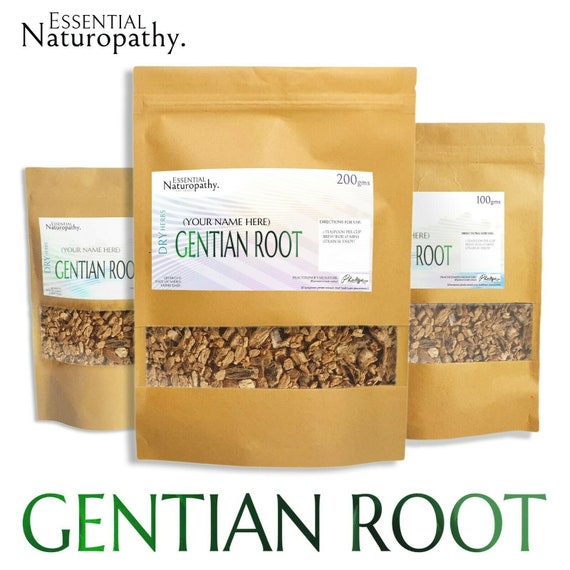The image showcases three beige, eco-friendly packaged food items labeled "Essential Naturopathy" with a simple design. Each package has a transparent window revealing the contents, which appear to be gentian root. The brand name "Essential Naturopathy" is clearly displayed at the top, followed by a placeholder text "Your Name Here," and the product name "Gentian Root" in blue text at the bottom. The largest package in the center is labeled 200 grams, while the sizes of the two smaller packages flanking the center are partially obscured, with one known to be 100 grams. The packaging also features a vertical label reading "Dry Herbs." The product photo highlights the rustic, natural appearance of the gentian root, which resembles mulch, set against a white background with subtle shadowing.